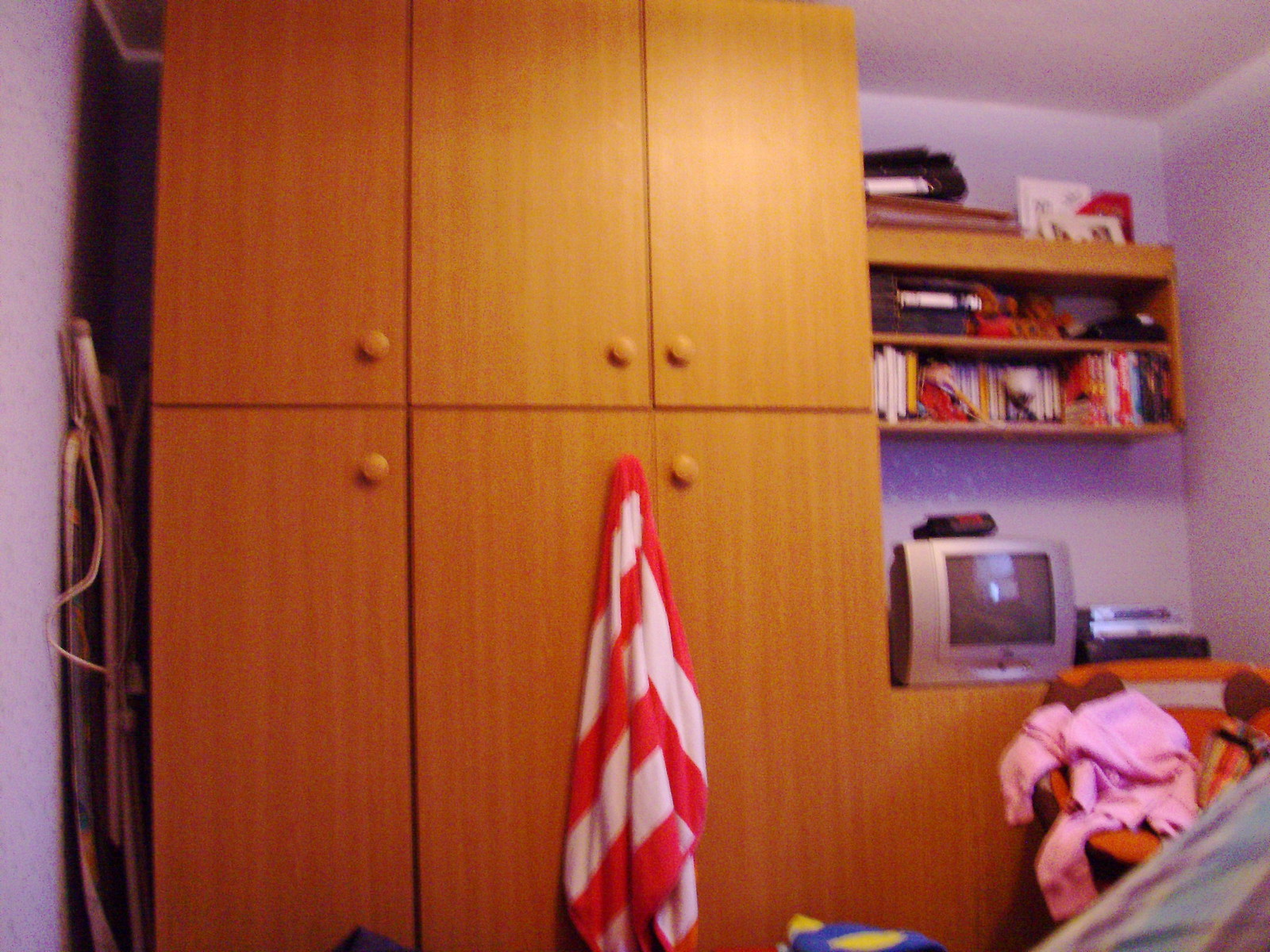The image depicts a dorm room or dorm room-like setting. It features a built-in furniture system made of light brown wood, including six storage lockers (three on top and three on the bottom) with large circular wooden handles. A red and white striped towel is hung on the middle bottom locker. Adjacent to this is a tabletop that holds a very small, old-style television with a silver exterior and a darker black screen. Stacked next to the TV are various books. Above the TV is a wooden shelf filled with colorful video cases in white, yellow, red, and blue. Toward the bottom right of the image, there is an orange chair adorned with a long-sleeved pink shirt. The furnishings in the room appear well-used and the area is somewhat cluttered with items scattered above the TV and on the chair.